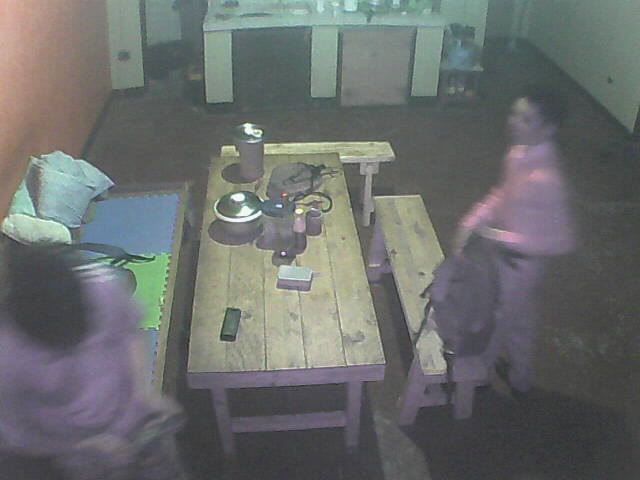The photograph captures a room with contrasting orange and white walls and a rustic ambiance highlighted by a handcrafted wooden table placed at the center, surrounded by matching wooden benches. The grain of the wood is visible, emphasizing its handmade quality. To the left, a low piece of furniture, possibly a bed, hosts three square mats and pillows at the end, partially obscured by a person with dark hair and a short-sleeved shirt, blurred as they hold an indistinct item. On the right, another person stands near the bench, facing sideways while wearing a pinkish shirt, tan pants, and black shoes, with a backpack placed on the bench. Both individuals have a slight motion blur, suggesting movement. The brown-carpeted floor adds warmth, contrasting with the countertop in the background, which features wooden details and various items on top. Adjacent to it, a smaller shelf and a doorway complete the backdrop, alongside what might be a black mini-fridge or dishwasher and a gray or white mini-fridge, tucked under the countertop.